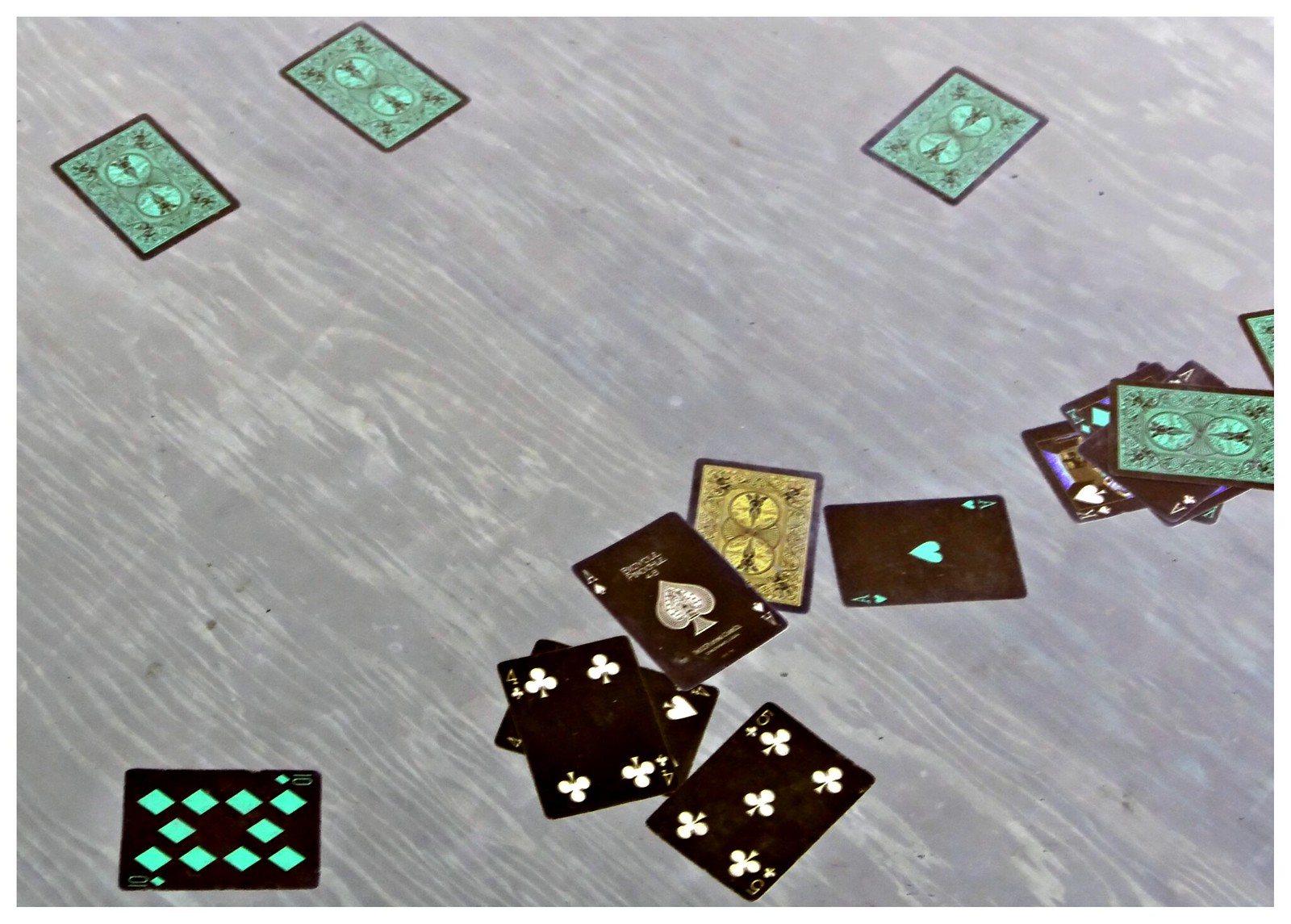A unique spread of playing cards features an unconventional color scheme, making the deck stand out. Each card has a black background, diverging from traditional designs. The numbers and suits are depicted in either a vivid green or stark white, contrasting sharply with the dark backdrop. Among the cards displayed, some are face up revealing an ace of hearts, an ace of spades, a five of clubs, and a ten of diamonds. Instead of standard red hearts, the ace of hearts showcases a green heart and a green 'A'. Similarly, the ace of spades maintains its iconic shape but in green, while typical black-suited cards like the five of clubs display white clubs and a white numeral '5'. This unusual palette adds an intriguing twist to an otherwise classic card game visual.